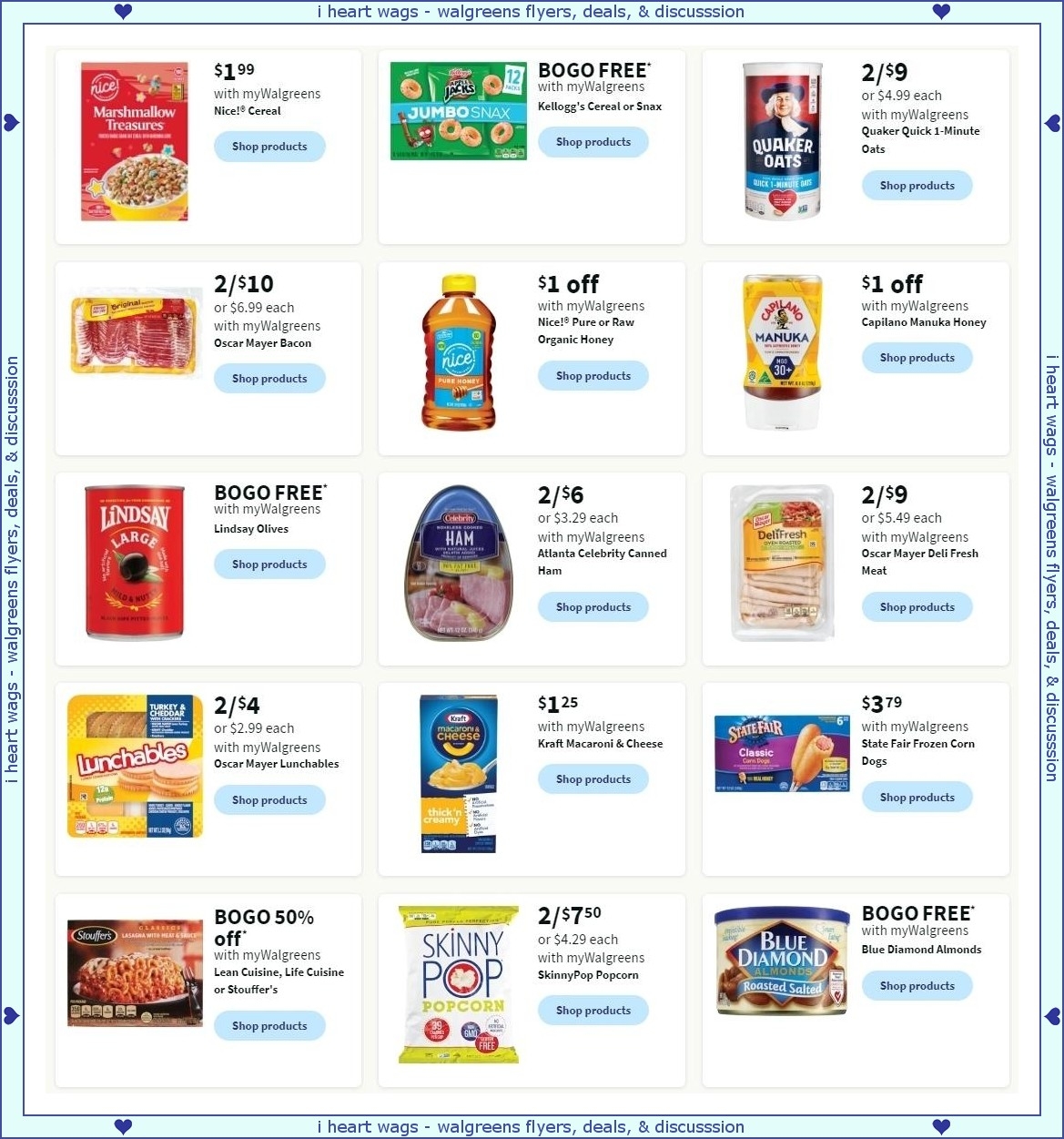**Detailed Caption:**

The image is a digital advertisement for groceries, designed as a nearly square white rectangle with a distinct light blue border. The border is intricately detailed, featuring very thin dark blue or black lines on both the inner and outer edges. This dual-line design delineates the stripe of light blue that encircles the entire square. Each side of the light blue border is adorned with small dark blue hearts – two on the top edge, two on the bottom edge, and two on each of the vertical edges. Between the hearts, the border is inscribed with the phrase "I ♥ Wags – Walgreens Flyers, Deals & Discussion" where ‘♥’ is a heart symbol and the word ‘and’ is represented by an ampersand.

Within this decorative border lies the main advertisement content, laid out in a grid format featuring five rows of products. Each row showcases three different items along with their associated deals and discounts.

- **Row 1** includes:
  - Marshmallow Toasty Cereal priced at $1.99 with MyWalgreens rewards.
  - A Buy One Get One Free offer for what appears to be a jumbo box of cookies.
  - A canister of Quaker Oats.

- **Row 2** presents:
  - Oscar Mayer Bacon available at two for $10.
  - An unspecified brand of organic honey with a $1 discount.
  - Another product with an unclear description but has a $1 discount.

- **Row 3** features:
  - Lindsay Olives available on a Buy One Get One Free promotion.
  - Danish Ham sold at two for $6.
  - Oscar Mayer Lunch Meat priced at two for $9.

- **Row 4** displays:
  - Lunchables at two for $4.
  - Kraft Macaroni and Cheese for $1.25.
  - State Fair Corn Dogs priced at $3.79.

- **Row 5** promotes:
  - Stouffer's entrees available at Buy One Get One 50% off.
  - Skinny Pop Popcorn priced at two for $7.50.
  - Blue Diamond Almonds on a Buy One Get One Free offer.

Each item listing includes its sale price or discount detail and a button labeled "Shop Products," likely indicating an option to add the item to an online cart.